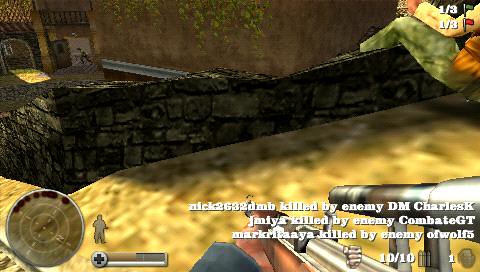This screenshot from a 1990s video game features a classic first-person shooter interface. On the right side of the screen, a hand holds a silver gun with a brown stock and barrel, equipped with a prominently mounted scope. In the upper left corner, a circular mini-map displays an 'X' and several dotted markers around its perimeter. The bottom left corner shows a health bar, which is approximately half depleted, alongside a gray silhouette of a figure holding a gun. 

The player stands on a brownish-green, tan surface that slopes downward towards a dark brick wall. In the middle distance, another character is visible in a walkway, with an archway to their left. Above the archway, a bridge or passageway is indicated. Further to the right, a wall adorned with vines or moss attests to the game's environmental details.

On the right side of the screen, near the gun, white text partially obscures the view, reading "Killed by enemy DM Charles." Alongside this, the game displays "10/10" ammo count and a numerical '1' in the corner, signifying either an in-game rank or score.